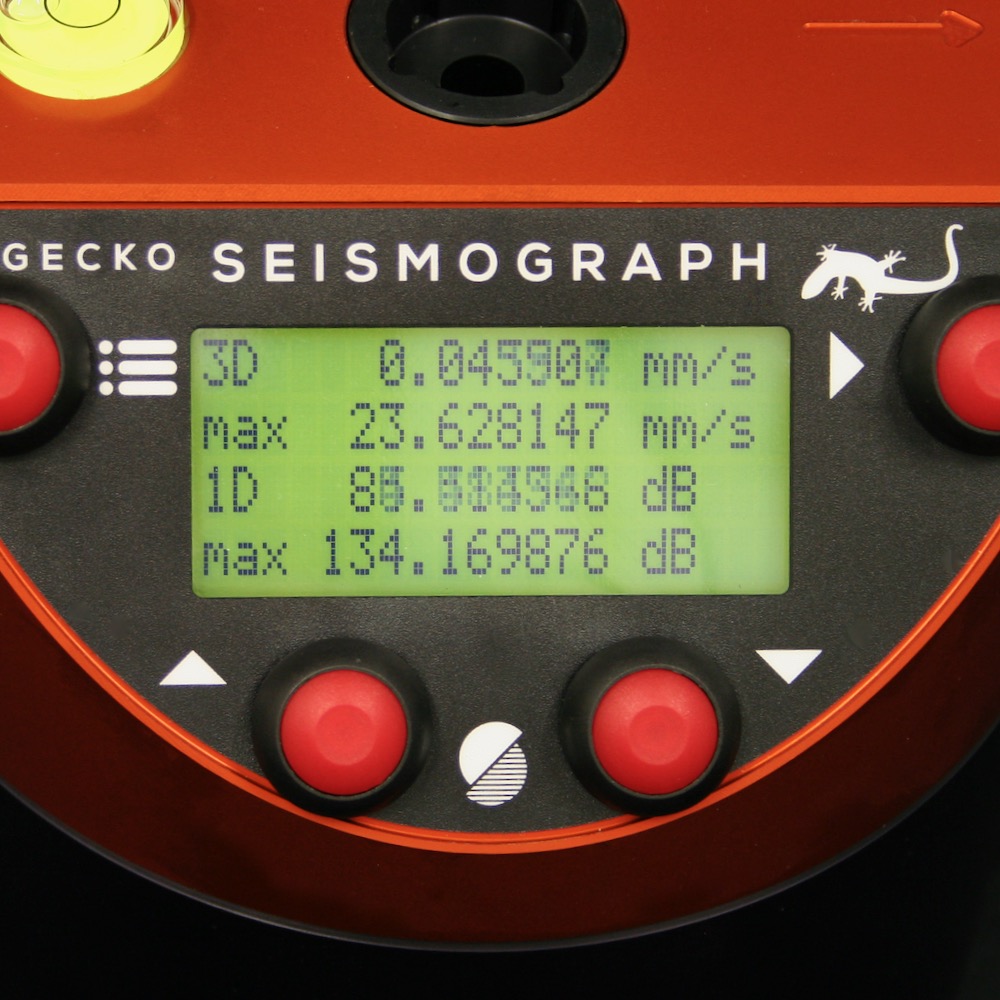This image is a close-up of a Gecko Seismograph, a black and red electronic device used for measuring seismic activity. The device prominently features a screen at the bottom surrounded by four red buttons—one on the left, two on the bottom, and one on the right. The screen displays four different measurements in a vertical list: "3D" measured in millimeters per second (0.045907 mm/s), "Max" also in millimeters per second (23.628147 mm/s), "1D" in decibels (85 dB), and "Max" in decibels (134 dB). Above the screen is the label "Gecko Seismograph" and next to it a logo featuring a graphic of a gecko. At the top of the device, there is a black hole presumably for plugging in accessories. The red buttons surrounding the screen control various functions of the seismograph, which aids in analyzing seismic data.